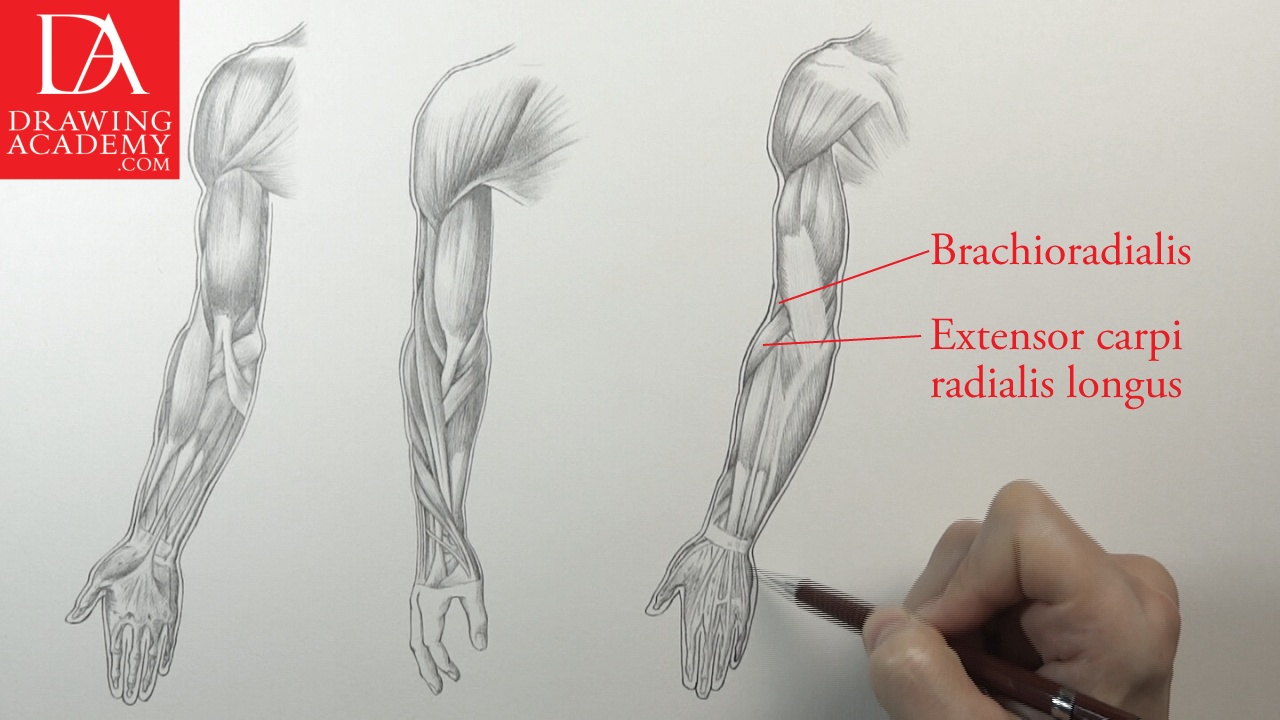The advertisement for thedrawingacademy.com features a detailed anatomical illustration of the human arm against a white background. In the bottom right corner, a right hand holding a mechanical pencil is actively drawing an intricate depiction of the arm's interior, revealing tendons and muscles. Three different versions of the arm illustration are displayed across the page, showcasing varying details and profiles. The far-right arm illustration is extensively labeled with red lines identifying specific muscles such as the brachioradialis and the extensor carpi radialis longus. To the left, the two additional arm illustrations present different views and details of the muscles and ligaments, with one arm revealing the palm and the other showing the hand in a different position. The top left corner of the image features a distinctive red box with the stylized, interlocking "D" and "A" logo, accompanied by the website name drawingacademy.com in white text.